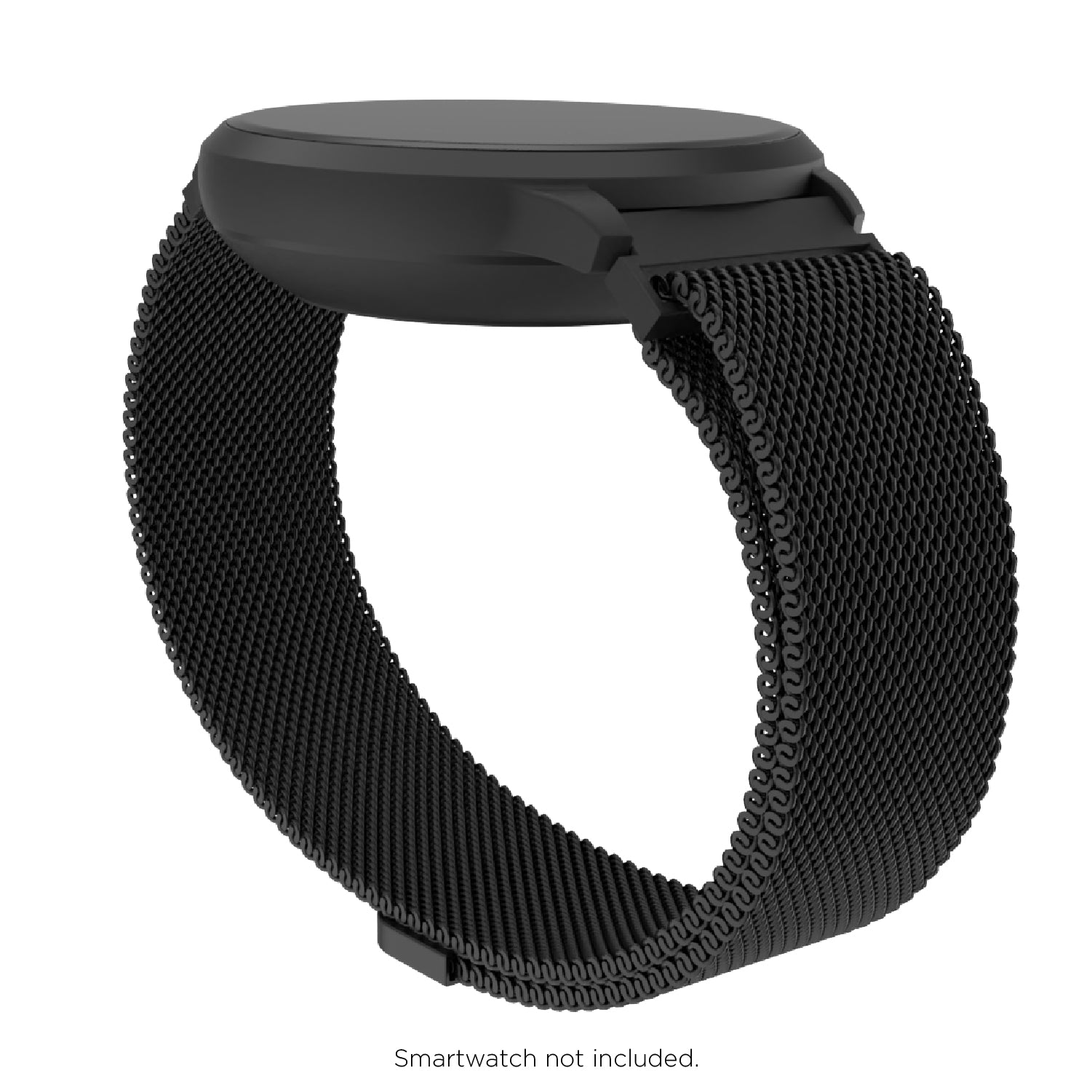The photograph showcases a sophisticated black wristwatch band with a shiny, circular interface. The sleek black band features a fine, well-defined cloth ribbon that allows for easy adjustment and secure fastening around the wrist. The background of the image is white, which highlights the dark, glossy appearance of the band. There's a noticeable tab at the bottom of the band, which is black and seemingly part of the adjustable mechanism. Additionally, the text at the bottom of the image reads "smartwatch not included," indicating that only the band is being sold. The overall design emphasizes a modern, minimalist aesthetic with its dark gray to black gradient and subtle, integrated styling elements.